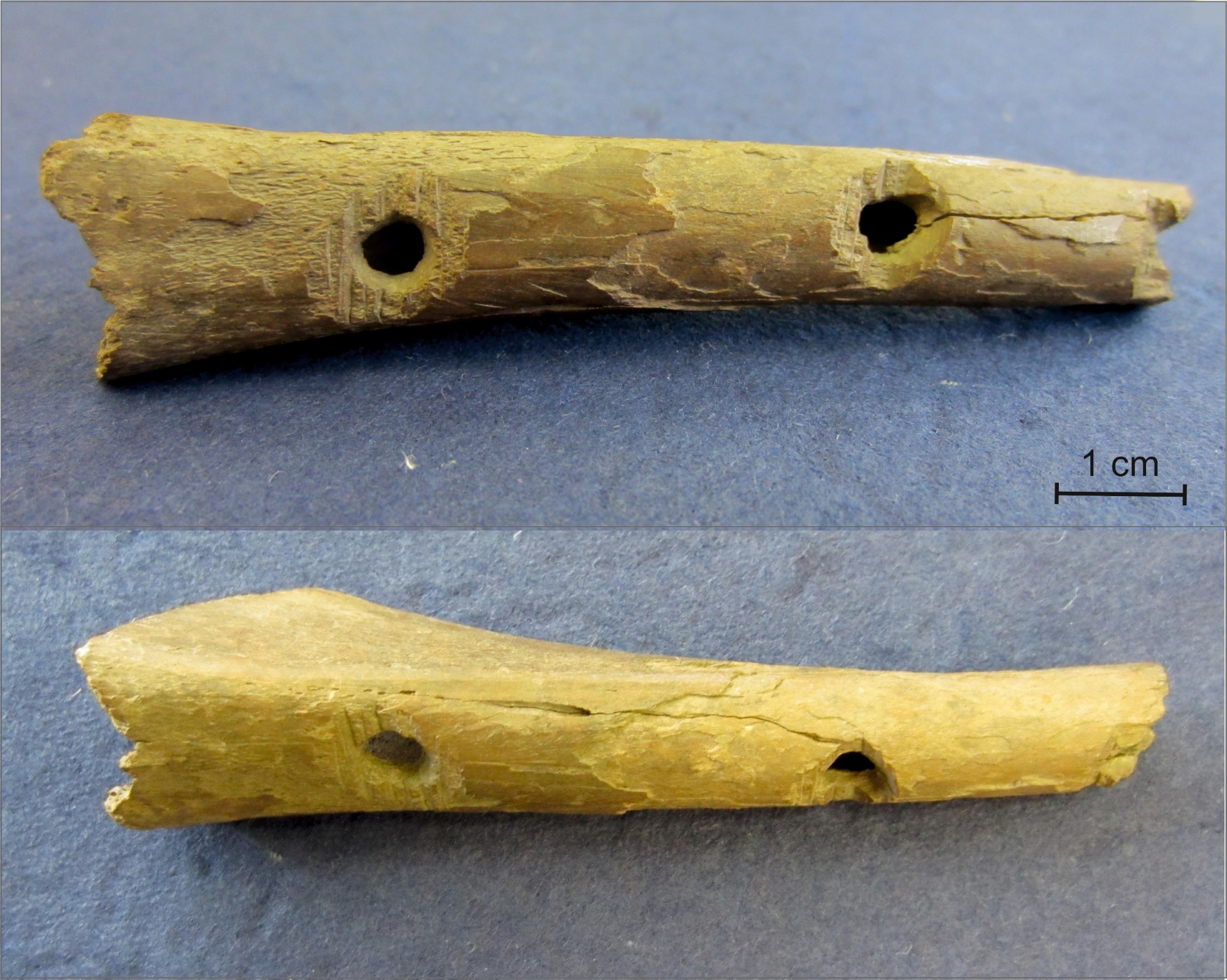The image consists of two color photographs, one above the other, showing the same object from different angles. The object appears to be a very weathered piece of wood, resembling a prehistoric flute or primitive instrument. Each photo captures the object positioned to the right. The wood has two holes carved out approximately three centimeters apart. A scale indicating one centimeter is visible in the image, providing a sense of size. The detailed texture and positioning suggest it is meant to be blown into, with one hole covered to produce sound.